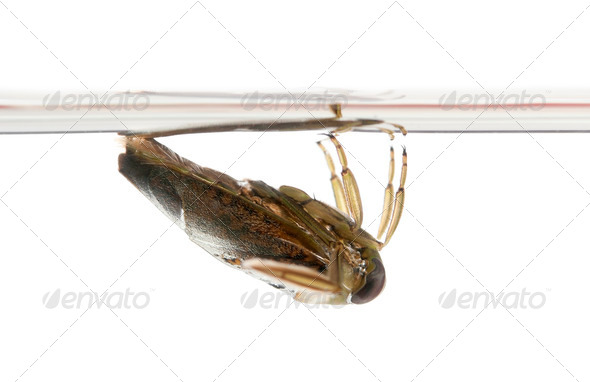This detailed image shows a dark brown insect, likely a moth, hanging upside down from a clear plastic tube, resembling a straw, which runs across the top third of the photo. The insect clings to the tube with four of its legs, and the base of its abdomen also touches the tube. Notably, the legs, mainly light brown and slightly translucent, appear to shimmer due to the bright lighting. The insect's folded wings are dark brown with black spots, reflecting some light. The background is stark white, enhancing the visibility of the insect and the thin tube. A watermark with the word "Envato" in a light gray crisscross pattern, repeating six times, overlays the image but doesn't obscure the main details.